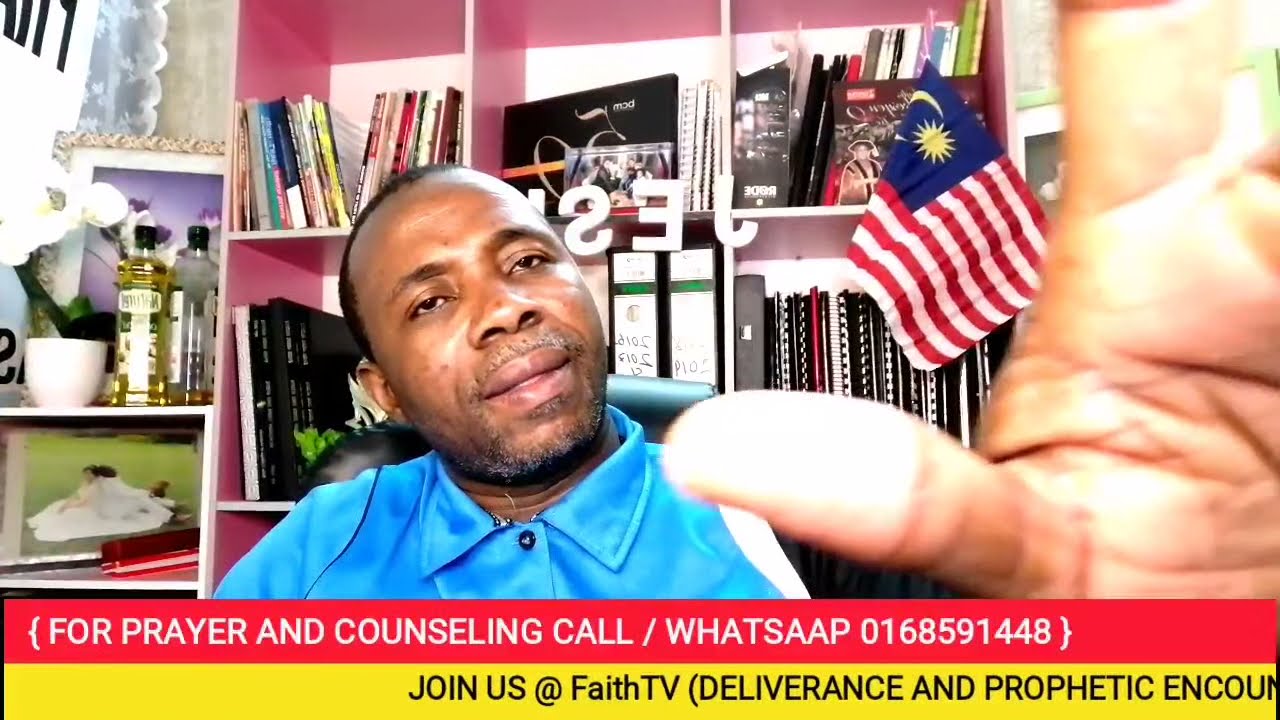In this detailed image, a Black man with short hair and light stubble, wearing a light blue collared button-up shirt, sits in a black leather office chair. His head is slightly tilted to the left, and his left hand is raised next to the screen, providing a close-up view of his thumb and part of his index finger, possibly as he adjusts the camera or tries to block it. His expression suggests concern or dissatisfaction, perhaps with the recording setup.

In the background, there is a pink and white bookshelf filled with hardcover books, spiral notebooks, and various manuals. To his right, another shelf houses plants and bottles that look like air fresheners. A distinctive flag resembling the American flag but with a sun and moon replacing the stars is visible on the bookshelf. The lower portion of the image features text banners; a prominent red banner reads, "For prayer and counseling, call WhatsApp 0168-591-448," and a yellow banner at the bottom indicates, "Join us at Faith TV Deliverance and Prophetic Encounter." The setting appears to be a normal room, potentially used for religious broadcasting or online evangelism.